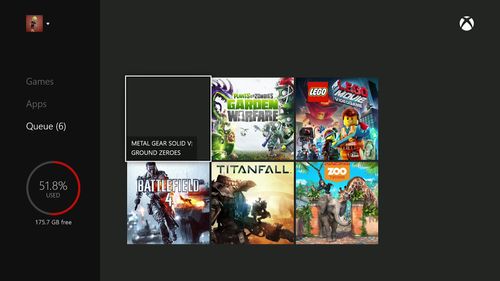A screenshot of a gaming dashboard, possibly from a PC or mobile device, showcasing various game management options. The interface features a vertical black column on the far left side, with a profile picture at the top followed by labeled sections: "Games," "Apps," and "Queue." The "Queue" section is highlighted, displaying a notification with "(6)" next to it. Below, a circular progress indicator shows "51.8% used" with "17% (7 GB) free."

In the central area of the dashboard, six game thumbnails are displayed in a grid layout. The games featured are:
1. Upper left: "Metal Gear Solid V: Ground Zeroes"
2. Upper middle: "Plants vs. Zombies: Garden Warfare"
3. Upper right: "LEGO® The LEGO Movie Videogame"
4. Lower left: "Battlefield"
5. Lower middle: "Titanfall"
6. Lower right: "Zoo Tycoon"